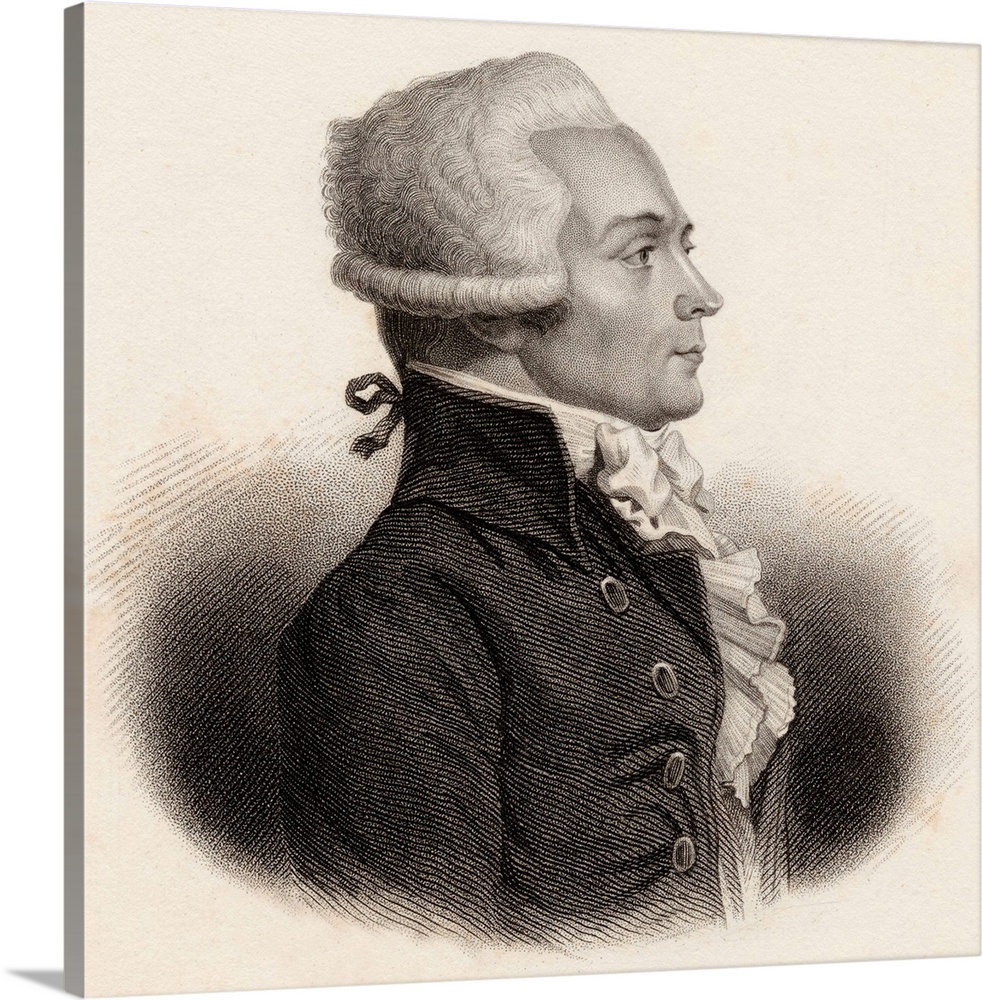This black-and-white hand-drawn portrait depicts a distinguished gentleman likely from the 17th or 18th century, possibly of English origin. The man features a white wig that reaches the middle of his ears with elegant curls framing his profile as he gazes leftwards, his lips pursed in a self-satisfied manner. His attire includes a tight-fitting black jacket adorned with four buttons and a high-collared white shirt with elaborate ruffles extending from his chin down to his chest. He has dark eyebrows and is encircled within a black oval on a plain white background, giving the portrait a classic and refined look, reminiscent of the Revolutionary War period.